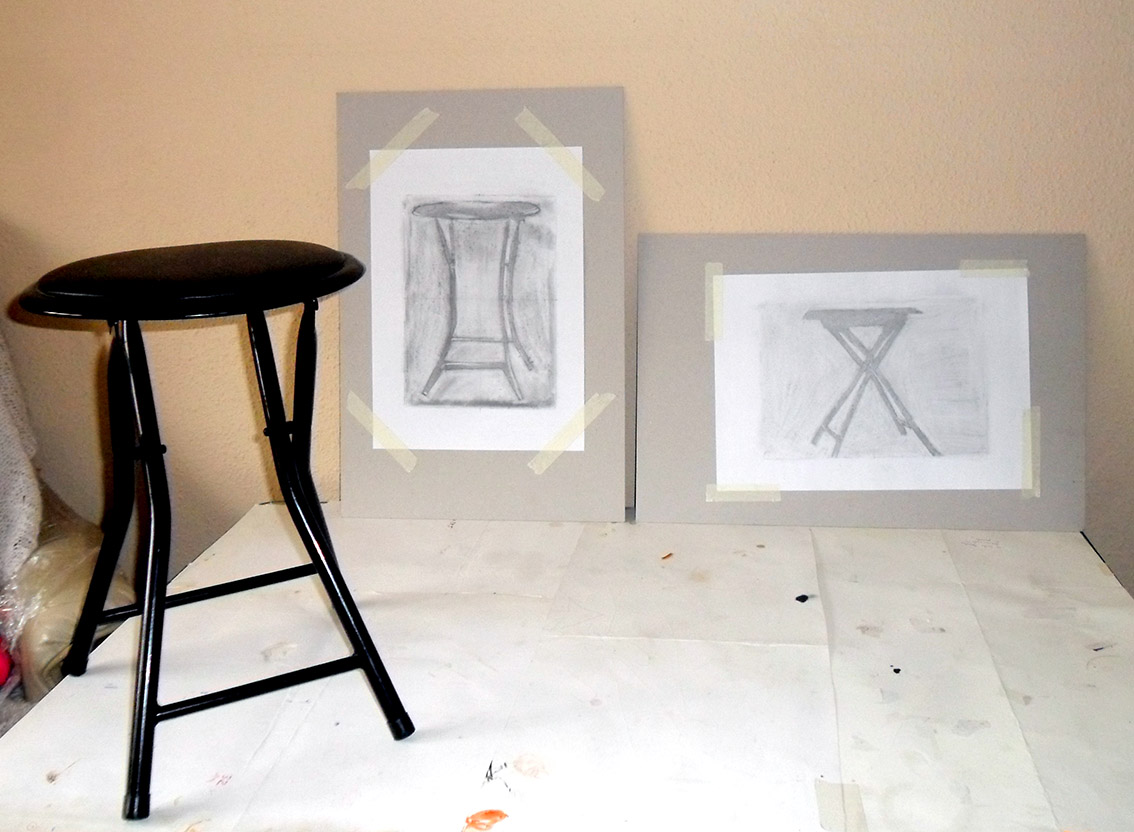This photograph captures a still-life setup showcasing a black metal stool, typically found in drawing classes, placed on a white platform. The platform, covered in overlapping pieces of white paper, appears somewhat haphazardly assembled, with some paper edges protruding. The stool is positioned on the left side of the image, in front of a beige plaster wall. Leaning against this wall are two charcoal or graphite drawings of the same stool, each mounted on larger pieces of paper using tape. The drawings depict the stool from different perspectives: the left drawing is in a taller, vertical (portrait) orientation, while the right drawing is in a wider, horizontal (landscape) orientation. This detailed arrangement emphasizes both the creative process and varying artistic angles captured in the sketches.